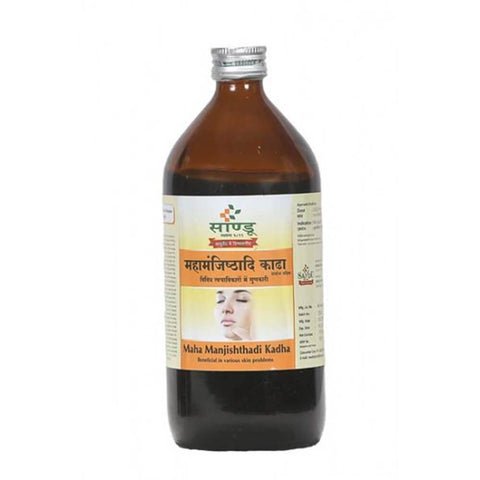This color photograph captures a brown, glass, medicine-style bottle with a silver screw-off cap, set against a clean white background. The bottle, filled with a dark liquid up to about four-fifths of its height, features a vibrant label dominated by yellow and orange hues. Central to the label is an image of a woman’s face, softly fading at the edges, as she gently rubs something into her chin with closed eyes, suggesting its use as a skincare product. The label displays a mix of design elements, including green text and two orange bands with black text, alongside a close-up of Indian-style writing that's mostly blurred and unreadable. The text at the bottom of the label, written in English, reads "Maha Maji Stadi Kadha." Above the image, there's a distinctive green and red logo accented with yellow squares and green diamonds. On either side of the central image, there's additional small, blurred text providing ingredient and product information.